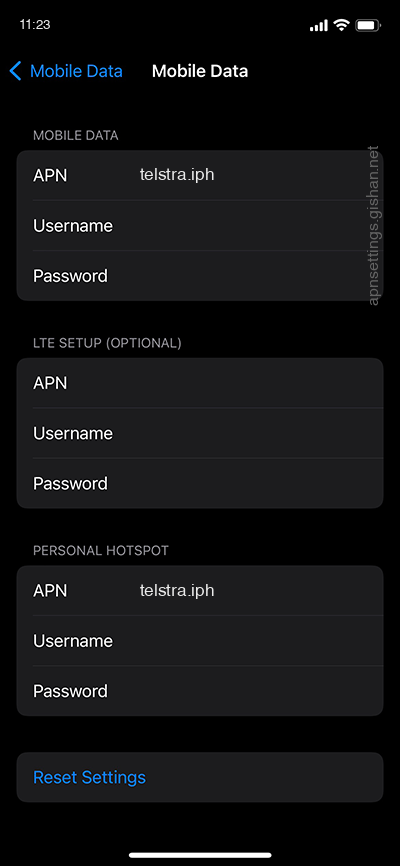### Phone Screenshot Details

The screenshot captures a section of the phone's mobile network settings at 12:21. The device displays full WiFi signal strength with four bars and has about 90% battery remaining.

#### Indicators
- **Top Bar**: 
  - **Time**: 12:21
  - **WiFi Signal**: 4 bars (full signal)
  - **Battery**: Approximately 90%

#### Mobile Data Settings
- **Indicators**: 
  - A blue arrow pointing left labeled "mobile data"
  - To the right, in white, the words "mobile data"
- **Blank Area**: 
  - Another instance of "mobile data"

#### Access Point Names (APN) Configuration
- **Grey Section**: 
  - **APN**: TLSTRA.IPH
  - **Username**: (blank)
  - **Password**: (blank)
- **LTE Setup (Optional)**
  - **Grey Section**: 
    - **APN**: (blank)
    - **Username**: (blank)
    - **Password**: (blank)

#### Personal Hotspot Settings
- **Black Header Section**: 
  - **Label**: Personal Hotspot
- **Grey Section**: 
  - **APN**: TLSTRA.IPH
  - **Username**: (blank)
  - **Password**: (blank)
  - **Button**: Reset Settings